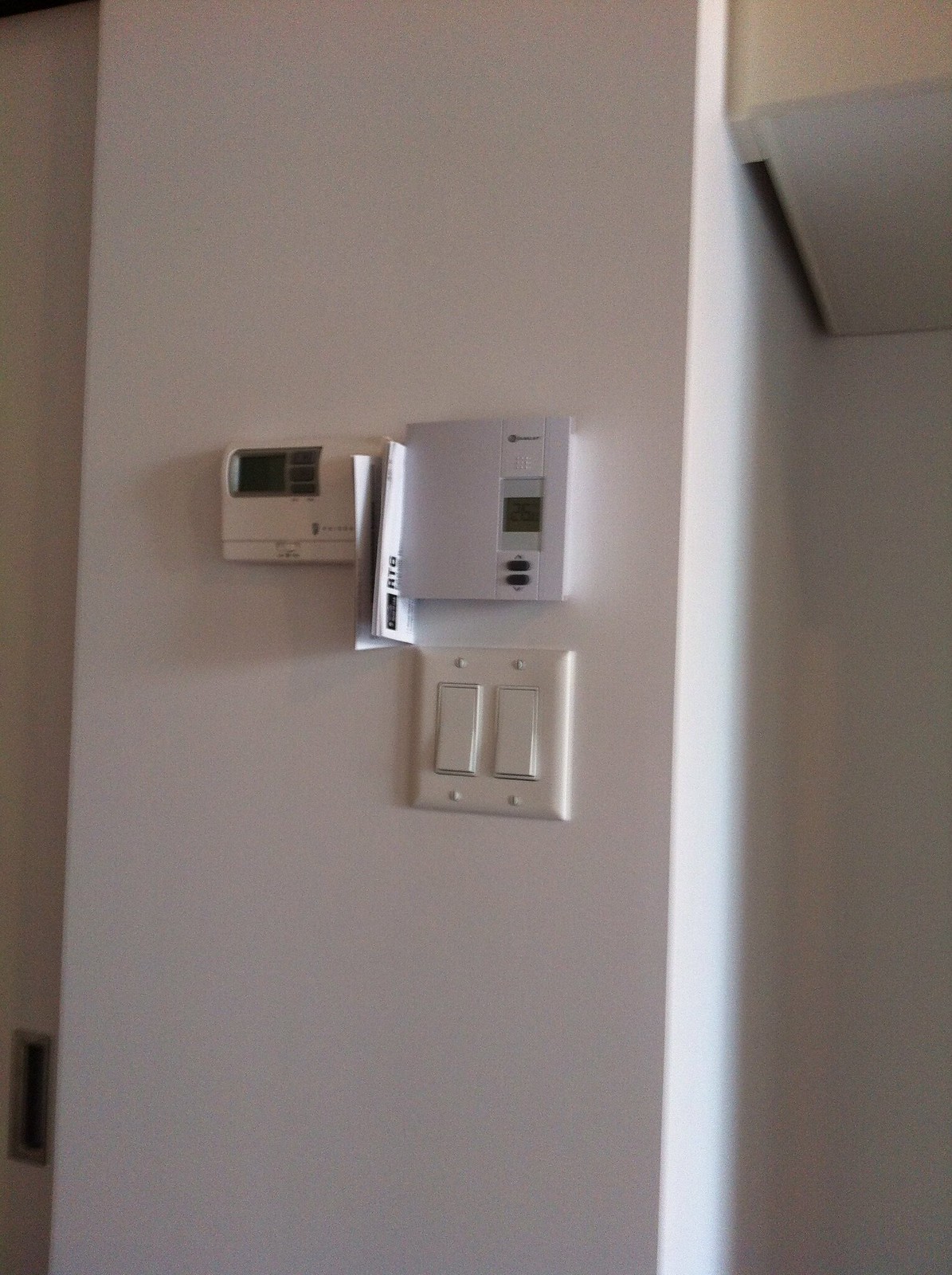A detailed photograph shows a white wall featuring two thermostats, a double light switch, and a ventilation grate. Centrally located is a tan double switch, secured by four screws positioned in pairs above and below each of the two switches. 

Above the switch is a modern, white thermostat with a small screen bordered by gray sections above and below. It has two black buttons on its interface. Next to this contemporary thermostat is an older, tan thermostat with a logo on its right side, which is partially obscured and difficult to read. The older device is characterized by larger buttons around its dated display, indicating it has likely been replaced by the newer thermostat.

Between the two thermostats is a folded piece of paper, possibly the installation instructions for the new thermostat. The paper is white with a black rectangle on top, inscribed with the indistinct lettering that appears to spell "RTEG." 

To the left of the thermostats and switches is a silver ventilation grate, contributing to the functional elements depicted in the image. The overall scene emphasizes the transition from old to new technology within the household setting.